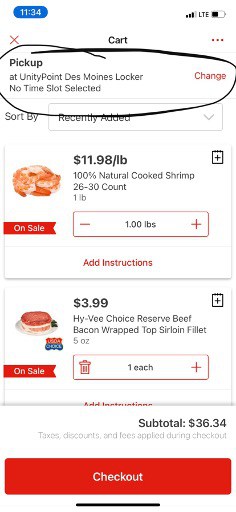The image is a screen capture from a mobile phone displaying a grocery delivery service app. At the top of the page, a header reads "Cart" with a red 'X' on the left-hand side for closing the page. Below this, the word "Pickup" is circled in black ink, followed by the location "Unity Point, Des Moines Locker," with no time slot selected. To the right of this text is a red button labeled "Change."

Further down, there's an option to sort items, with a dropdown menu currently set to "Recently Added." Below, there are two food items visible on the screen:

1. The first item is shrimp, shown with an image on the left. To the right, the price is displayed along with the title "Shrimp." The quantity selected is 1 pound, with buttons available to increase or decrease the amount. Below this, a small red button labeled "Add Instructions" is present.

2. The second item is a "Beef Bacon-Wrapped Sirloin Fillet," with an image on the left and the price of $3.99 displayed. The item weight is 5 ounces, and there are icons to delete or adjust the quantity. The quantity selected here is 1.

At the bottom of the page, the subtotal is shown as $36.34, along with a prominent red button labeled "Check Out."